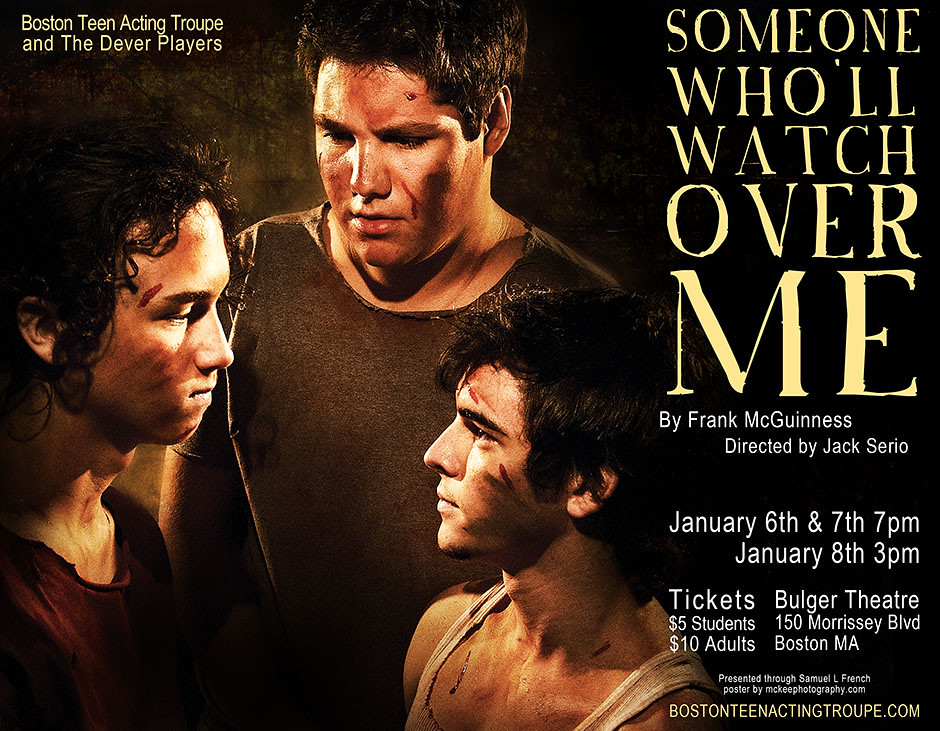The event poster features a predominantly black background that transitions into a dark brown hue. On the left side, three young men, appearing battered with sweat, bloodstains, and cuts, are depicted in a tense standoff. One of them is dressed in a dark t-shirt while another wears a dark shirt showing scuff marks on his face. The mood is intense as they glaringly confront each other. In the upper left corner, in yellow text, it reads "Boston Teen Acting Troop and the Deaver Players." Dominating the right side of the poster, bold yellow capital letters announce the play title "SOMEONE WHO WILL WATCH OVER ME," with credits below in white text: "by Frank McGinnis, directed by Jack Serio." The performance dates are listed as January 6th and 7th at 7 p.m., and January 8th at 3 p.m. The venue is the Bulgee Theater, located at 150 Morrissey Boulevard, Boston, Massachusetts. Ticket prices are indicated as $5 for students and $10 for adults. At the bottom, additional information states "presented through Samuel L. French" and credits "poster by McKeePhotography.com." The Boston Teen Acting Troop's website, BostonTeenActingTroop.com, is prominently displayed for further details.